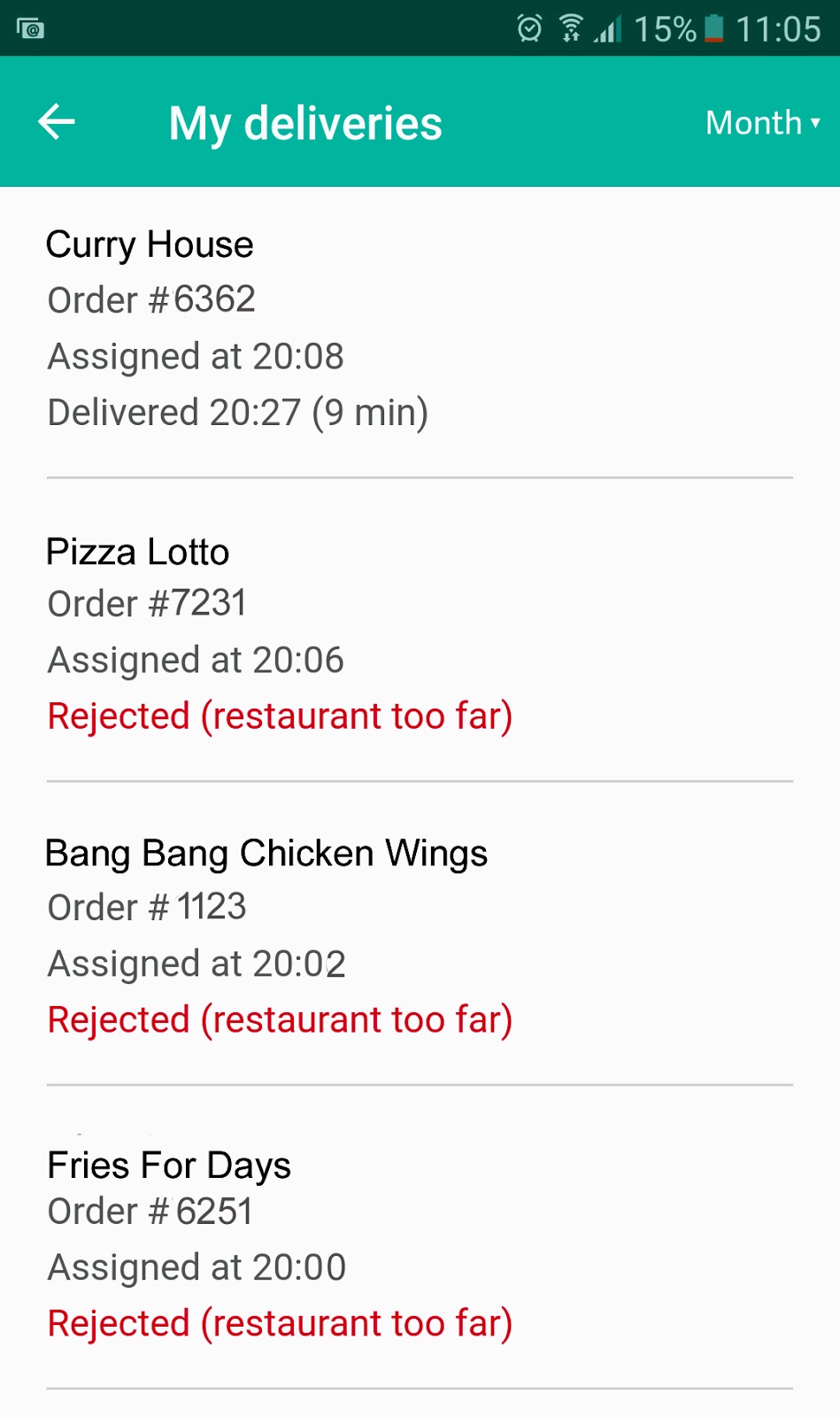The image displays a mobile phone interface, likely on an Android device, showcasing the delivery order history from a food delivery app. At the top, a banner with the text "My Deliveries" in white sits against a teal background, with an option to select the month on the right-hand side.

In the detailed breakdown, the delivery history lists various orders, including those that were rejected due to the restaurant being too far. This interface seems to be designed for a delivery driver, providing information on assigned and delivered orders, as well as reasons for rejections.

The most recent entry at the top shows a delivery from "Curry House" assigned at 8:08 PM (order number 6362) and delivered at 8:27 PM, indicating a delivery time of 9 minutes. Below this, several rejected orders are listed:

- "Fries for Days," assigned at 8:00 PM.
- "Bang Bang Chicken Wings," assigned at 8:02 PM.
- "Pizza Lotto," assigned at 8:06 PM.

Each rejected order notes the assignment time and the reason for rejection, contributing to a comprehensive overview of the driver’s delivery activity and rejections for that period.